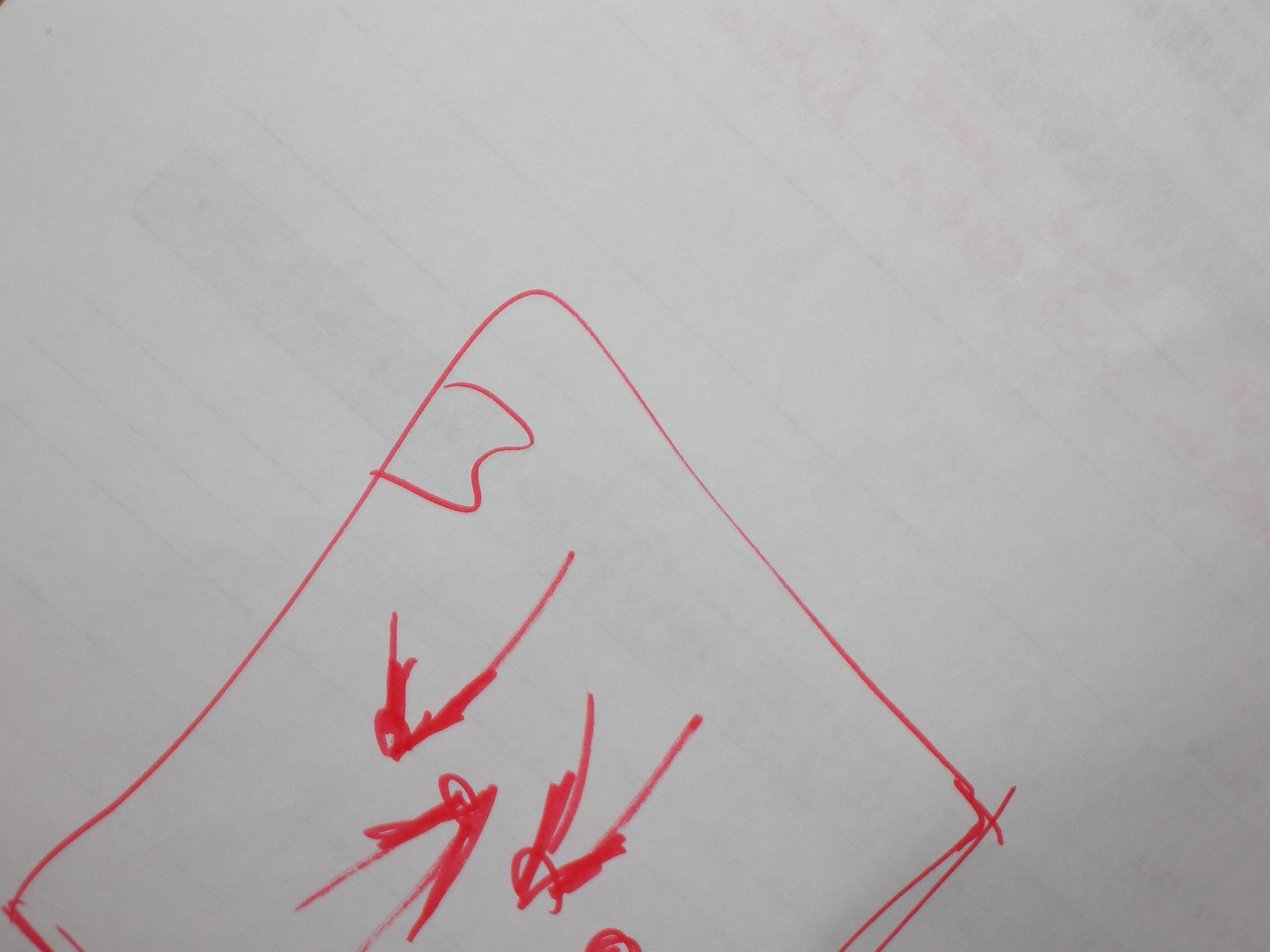In the photograph, there is a piece of wide-ruled notebook paper, distinguished by light blue horizontal lines. The focal point of the image is a drawing towards the bottom, executed with a thin-tip red marker. At first glance, the drawing appears to depict an 'M' character, positioned close to the edge of the paper, giving the impression of an enclosed area. This drawing is bordered by a red frame encompassing the entire picture.

Within the drawing, there are multiple markings resembling the letter 'V' or checkmarks; some are oriented upside down, while others face different directions. These marks might symbolize heads, possibly with hair, suggesting the depiction of human figures. There seem to be three complete figures alongside an additional, partially cut-off image on the right edge of the frame.

On the right side, there is an attempt to draw another frame, with overlapping lines creating an 'X' in the corner, accentuating the boxed layout of the artwork.